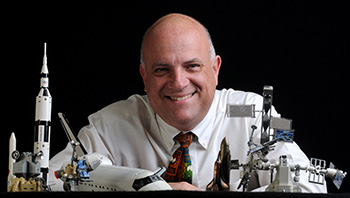The photograph features a smiling, balding man in his late 50s or early 60s, with a hint of gray hair on the sides of his head. He is dressed in a white long-sleeved collared shirt and a patterned tie, which includes colors such as red, blue, green, and possibly orange. The man also appears to be wearing a watch. He is seated against a completely black background, which highlights the models of various space-related objects positioned in front of him. Directly in front of him is a model of a large white rocket with black design trim. To the left of this rocket is a black and white space shuttle with a pointed tip. Near this, there appears to be a setup resembling an international space station with small attached satellites and spacecraft. Additionally, on the right side of the image, there are more models of rockets, satellites, and other space travel elements, primarily in shades of gray. The overall scene gives an impression of a knowledgeable individual surrounded by symbols of space exploration.